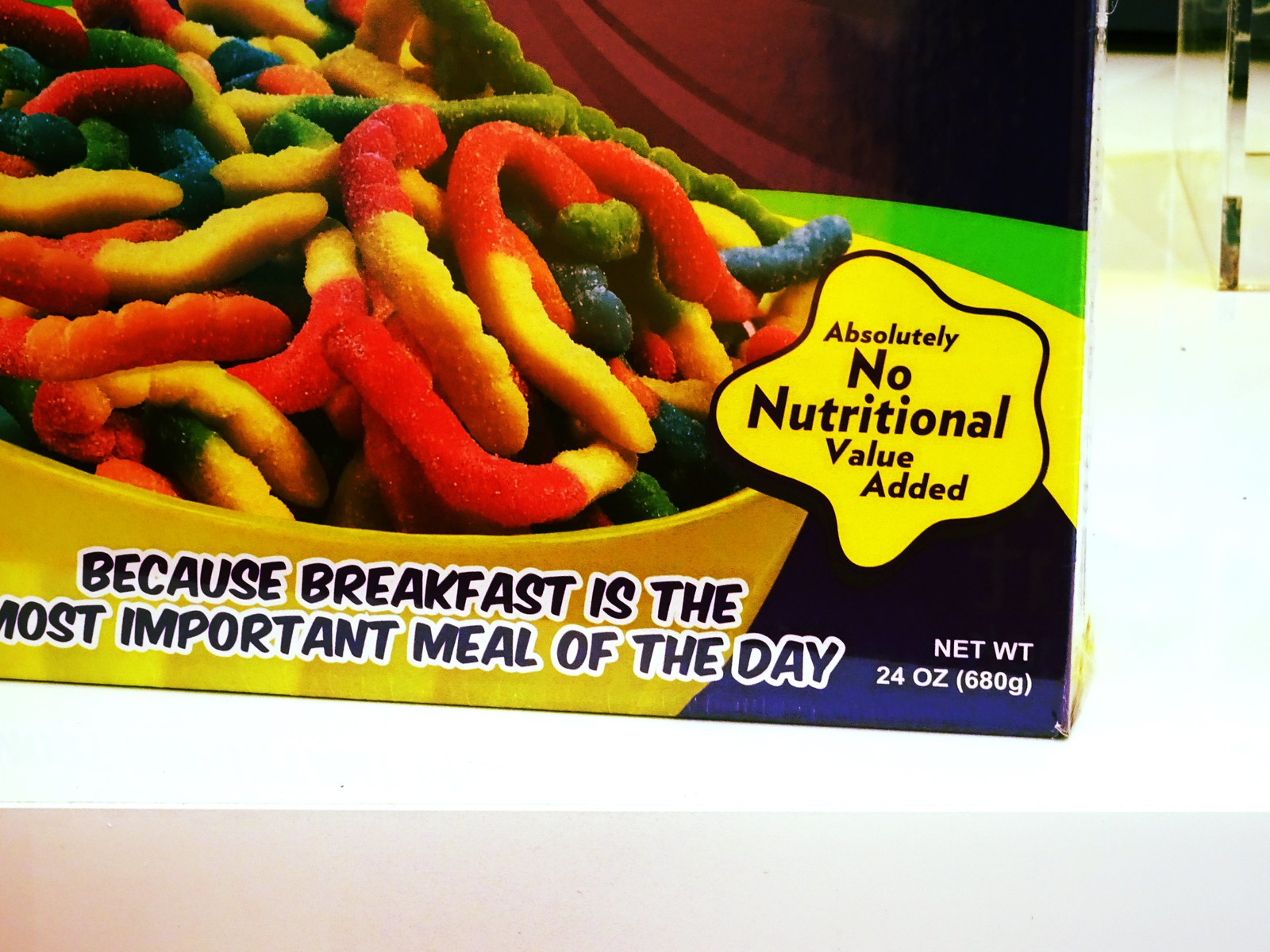A bright yellow plastic bowl brimming with an assortment of colorful gummy worms—yellow, orange, green, and blue—takes center stage in this vibrant image. The bowl, seemingly lifted from a playful advertisement, is set against a clean, neutral background. To the right of the bowl, a whimsical yellow cloud bordered in black contains the humorous disclaimer: "Absolutely no nutritional value added." Bold black text, outlined in white, stretches across the bottom of the image, proclaiming with a tongue-in-cheek tone: "Because breakfast is the most important meal of the day." The overall scene combines vivid colors and playful fonts to create an eye-catching, satirical take on breakfast advertising.